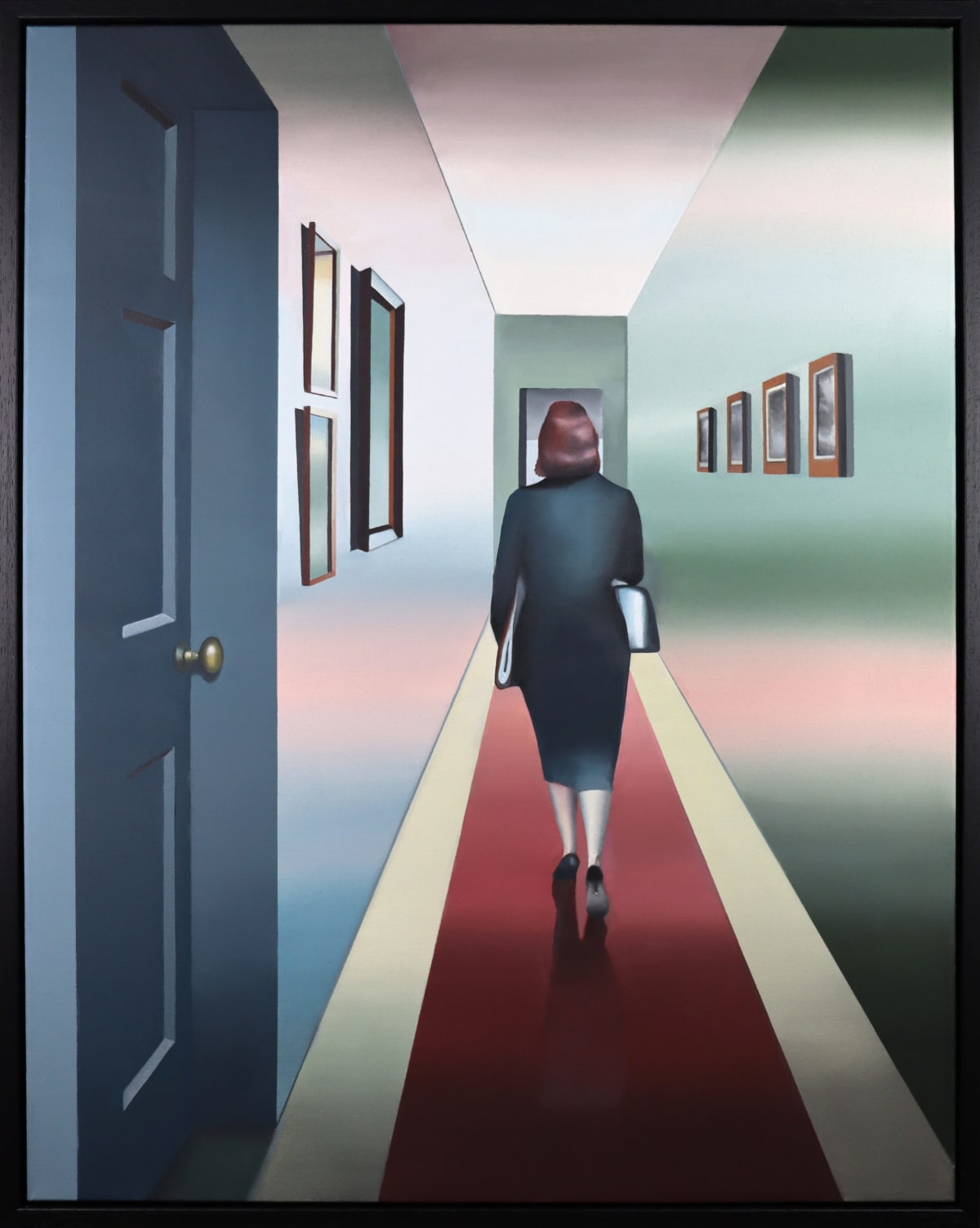This is a detailed illustration by Hogan Brown depicting a woman walking away from the viewer down a narrow hallway. The woman has shoulder-length brown hair and is dressed in a dark blue dress with black high-heeled shoes. She carries a bag under her right arm and some papers under her left arm. The hallway floor features a central red carpet strip, while the remaining floor space is a combination of green and tan hues.

The walls of the hallway exhibit a striking color gradient, where the left wall transitions from blue to a reflective pink, and the right wall transitions from green to a similar pink hue. The left wall, primarily blue, has a mix of one large photo and two smaller ones framed and aligned vertically. The right wall, predominantly green, displays a row of four black-and-white photos framed in brown, arranged to form a square pattern.

In the immediate foreground on the left, there is a large blue door with a brass doorknob. The hallway culminates in an open door at the far end, inviting the viewer’s gaze further into the composition. The entire scene is bordered by a black frame, adding a sense of closure to this visually intricate setting.